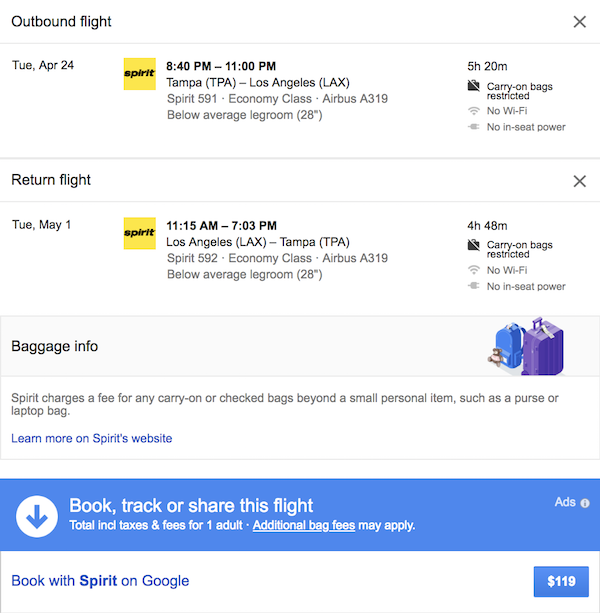The webpage offers details for booking a round-trip flight from Tampa (TPA) to Los Angeles (LAX) with Spirit Airlines. 

**Outbound Flight:**
- **Date:** Tuesday, April 24th
- **Departure Time:** 8:40 PM
- **Arrival Time:** 11:00 PM
- **Travel Duration:** 5 hours, 20 minutes
- **Flight Details:** Spirit Airlines Flight 591, Economy Class on Airbus A319
- **Amenities:** Below average legroom (28 inches), no WiFi, no in-seat power
- **Baggage Info:** Carry-on bags are restricted

**Return Flight:**
- **Date:** Tuesday, May 1st
- **Departure Time:** 11:15 AM
- **Arrival Time:** 7:03 PM
- **Travel Duration:** 4 hours, 48 minutes
- **Flight Details:** Spirit Airlines Flight 592, Economy Class on Airbus A319
- **Amenities:** Below average legroom (28 inches), no WiFi, no in-seat power
- **Baggage Info:** Carry-on bags are restricted

Below the flight options, the page provides Spirit Airlines' baggage policy details. At the bottom, there is a blue bar with options to book, track, or share the flight along with a prompt to book with Spirit on Google at a price of $119.